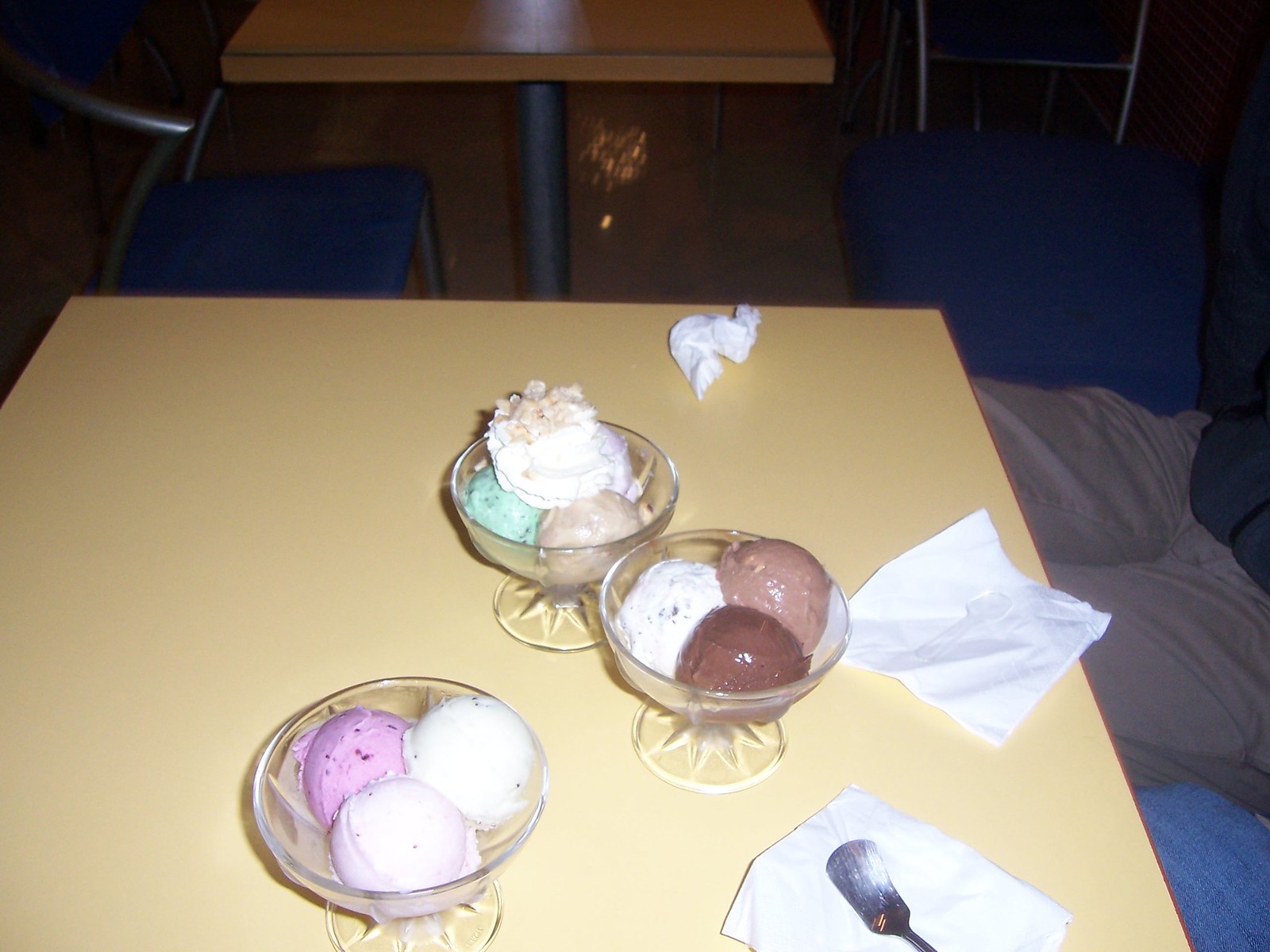This is a detailed photograph taken in what appears to be a cafeteria or a restaurant. The scene features multiple yellow square-topped tables, each supported by metal poles fixed to a shiny, light-colored linoleum floor. Surrounding the tables are royal blue chairs with metal arms and legs, and metal backrests. In the foreground, two individuals are seated to the right; one wears blue jeans visible at the knee, while the other sports a black top and gray pants.

Prominently displayed on the yellow table in the forefront are three white plastic bowls of ice cream, each with flared bases. The front bowl contains two white scoops and a pink scoop. The middle bowl, to the top right of the first, holds a white scoop with black chunks, a light brown scoop, and a dark brown scoop. The third bowl, positioned to the top left of the middle one, includes a white scoop—possibly with nuts—a light brown scoop, and a mint green scoop. 

Also on the table are three napkins—two intact and one crumpled—as well as a silver, shovel-shaped ice cream spoon placed on one of the napkins. In the background, more yellow tables and blue chairs are visible, suggesting the setting is a communal dining area like an ice cream cafe. The rightmost portion of the image shows a couch-like seating area with gray seats and blue or white pillows, reinforcing the casual, welcoming atmosphere of the establishment.